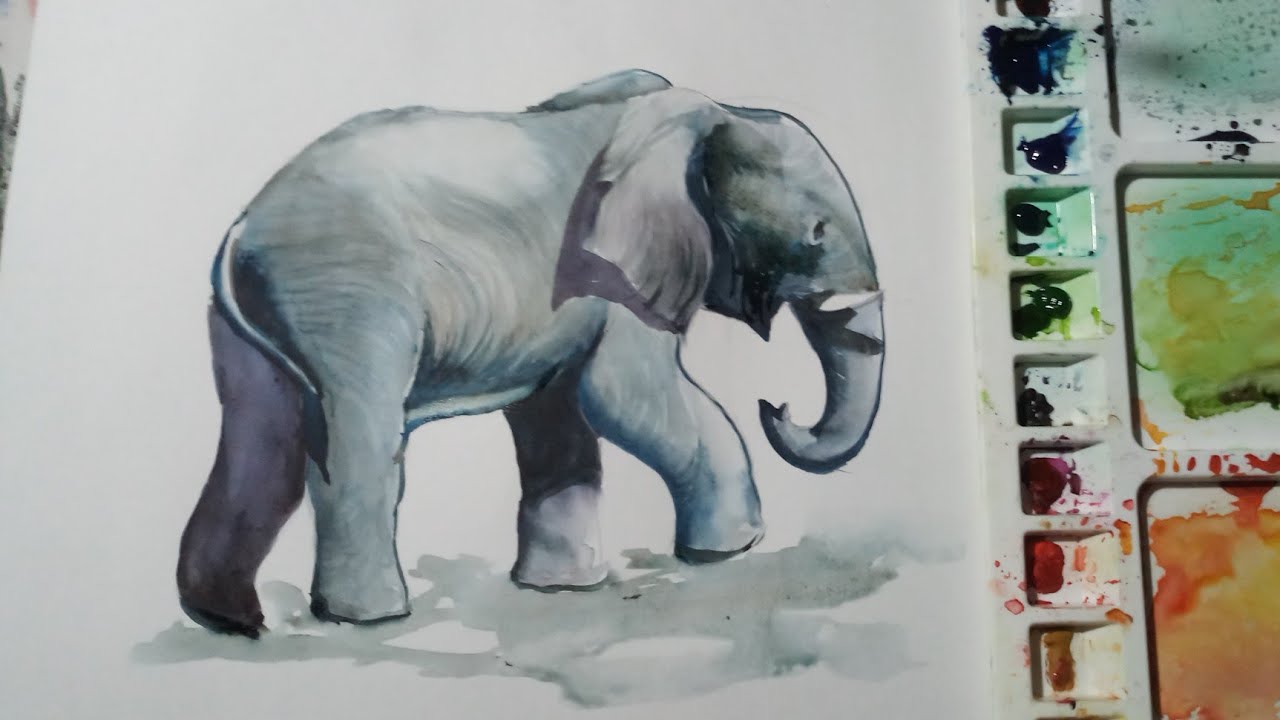This detailed watercolor painting captures a side profile of an elephant, which is primarily rendered in various shades of gray. The artwork is presented on a white paper background, with the elephant oriented to the right and appearing in mid-stride, its head slightly tilted upwards. The trunk hangs down but curls back towards the mouth, and a single tusk is visible on the right side. The elephant's ears rest gently by its side, contributing to its soft, curved appearance, possibly suggesting it's a young elephant.

On the right-hand side of the image, there is a visible, somewhat messy art palette, showcasing remnants of paint used in the artwork. The palette features small grooves in a white plastic container, indicating where the paint, in colors like orange, pink, purple, green, teal, red, and yellow, was accessed or mixed. Most of these colors have been used up, leaving only remnants behind. This careful arrangement of colors and their application suggests a professional and meticulous artistic process, emphasizing the detail and care taken in creating the painting. The overall image exudes a sense of artistic dedication and craftsmanship.